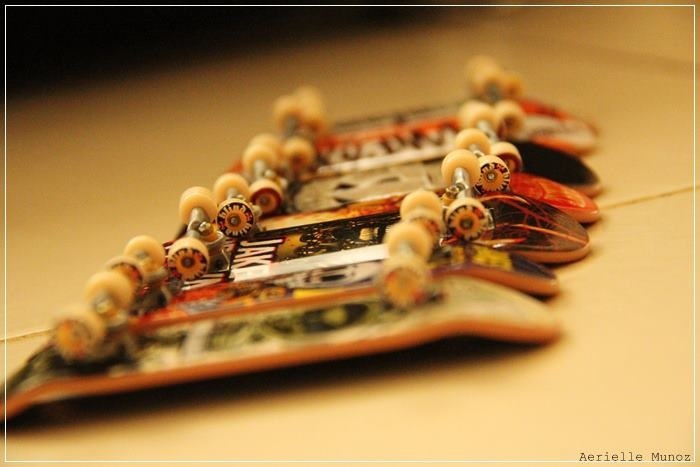This semi-professional photograph, taken by Ariel Munoz, features a close-up of miniature toy skateboards arranged indoors, possibly on a linoleum or tiled surface. The boards are oriented upside down, showcasing their wheels, which are predominantly orange, white, and red. The skateboards are tightly nestled side by side in a diagonal alignment, creating a vibrant array of colors from the various designs, logos, sponsors, and graphic images decorating their undersides. The entire setup forms a visually striking jumble of hues, including yellow, orange, black, white, and red. A thin white frame encapsulates the image, with one skateboard extending slightly out of frame. The photographer's watermark is clearly visible in the bottom right corner, adding a professional touch to the scene.